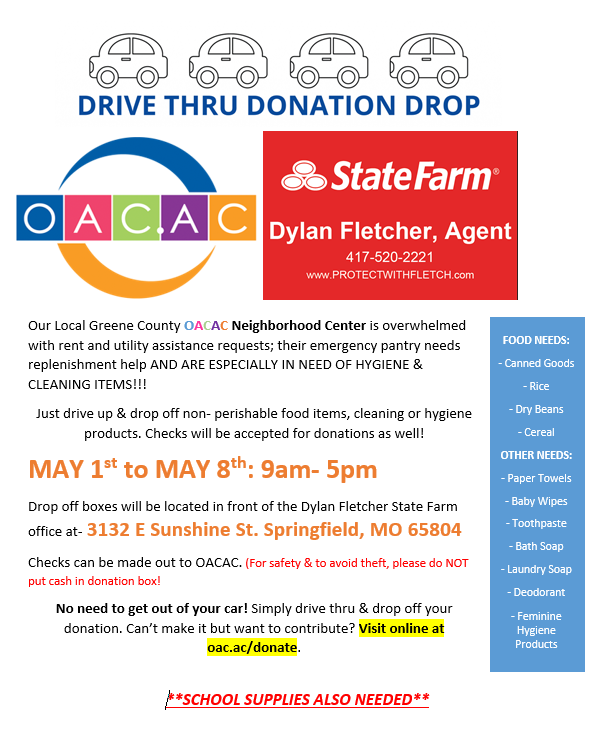This advertisement for a donation drive is set against a plain white background and features a variety of detailed sections. At the top of the image, there are cartoon outlines of four cars. Below these cars, large blue text reads "Drive-Thru Donation Drop." Beneath this headline, on the left, there is a logo for OACAC, a neighborhood center, presented as a circle divided in half with blue on the top and orange on the bottom, spelling out "OACAC" in colorful squares with white letters. To the right, a red rectangle with white text displays "State Farm, Dylan Fletcher, Agent 417-520-2221, www.protectwithfletch.com."

Below these logos, black print provides a detailed description of the donation drive, explaining that the Greene County OACAC Neighborhood Center is overwhelmed with rent and utility assistance requests, and urgently needs hygiene and cleaning items. Instructions follow, stating that non-perishable food items, cleaning, or hygiene products can be donated by simply driving up and dropping them off. The donation event runs from May 1st to May 8th, from 9 a.m. to 5 p.m., with boxes located in front of the Dylan Fletcher State Farm office at 3132 East Sunshine Street, Springfield, Missouri, 65804. Additionally, checks can be made out to OACAC, but cash should not be deposited to avoid theft. For those unable to attend, online contributions can be made through the highlighted URL, oac.ac/donate.

On the lower right, a vertical blue rectangle with white text lists specific donation needs: canned goods, rice, dry beans, cereal, paper towels, baby wipes, toothpaste, bath soaps, laundry soap, deodorant, and feminine hygiene products. Orange text emphasizes the event dates and location details, ensuring clarity. Finally, a red note with asterisks highlights that school supplies are also needed.